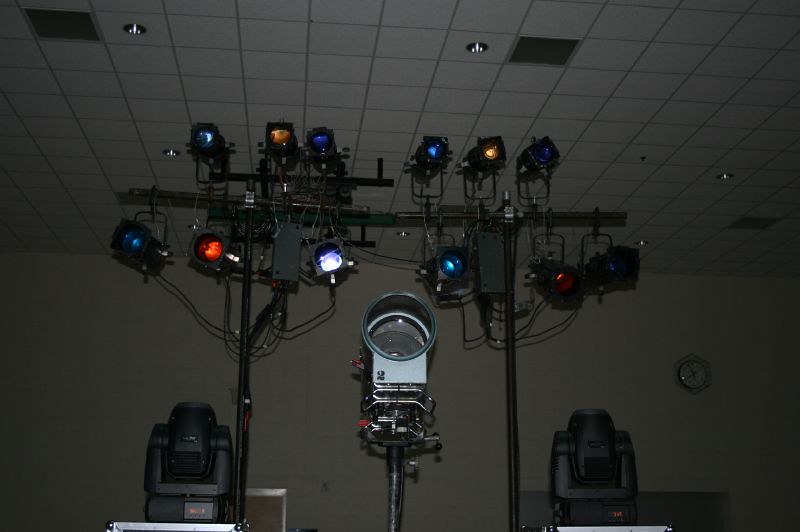The image is set inside a darkened studio room with a white tiled ceiling featuring two small silver circle lights and square air vents. The walls are a tan color, slightly darker than the ceiling. The room is equipped with two black poles supporting multiple studio lights arranged in two sets. Each pole has three lights at the top and three at the bottom, displaying various colors including teal, yellow, dark blue, medium blue, red, orange, purple, and lighter blue. Wires from the lights hang down, adding to the studio feel. In the center of the image stands a significant spotlight with a big round head and a square base on a black pole, adorned with more wires, buttons, and knobs. There is also a wide lens, possibly a camera, situated on a black stand. A small clock can be seen on the right side of the wall.